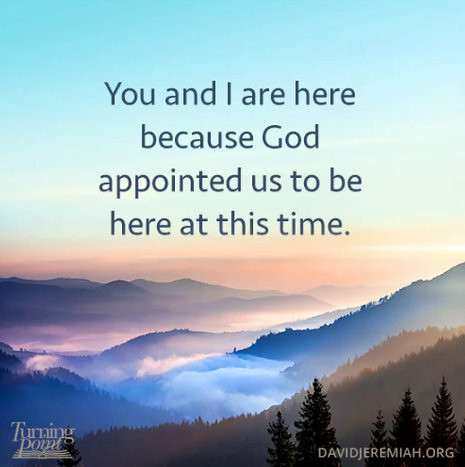The image is a detailed, square-format color illustration that combines fantasy-style artwork with an inspirational message. The lower half depicts a serene, forested mountain landscape at sunrise, with brown and green pine trees in the foreground. The mid-ground features a blue mountain range enveloped in white clouds, flanked by a purple mountain range in the distance under a pink sunrise. Low-lying fog enhances the ethereal atmosphere between the hills. The upper half of the image transitions into a light blue morning sky, onto which black text is superimposed, stating, "You and I are here because God appointed us to be here at this time." The bottom left corner holds a white logo of an open book reading "Turning Point," while the bottom right corner displays "DavidJeremiah.org" in white text.